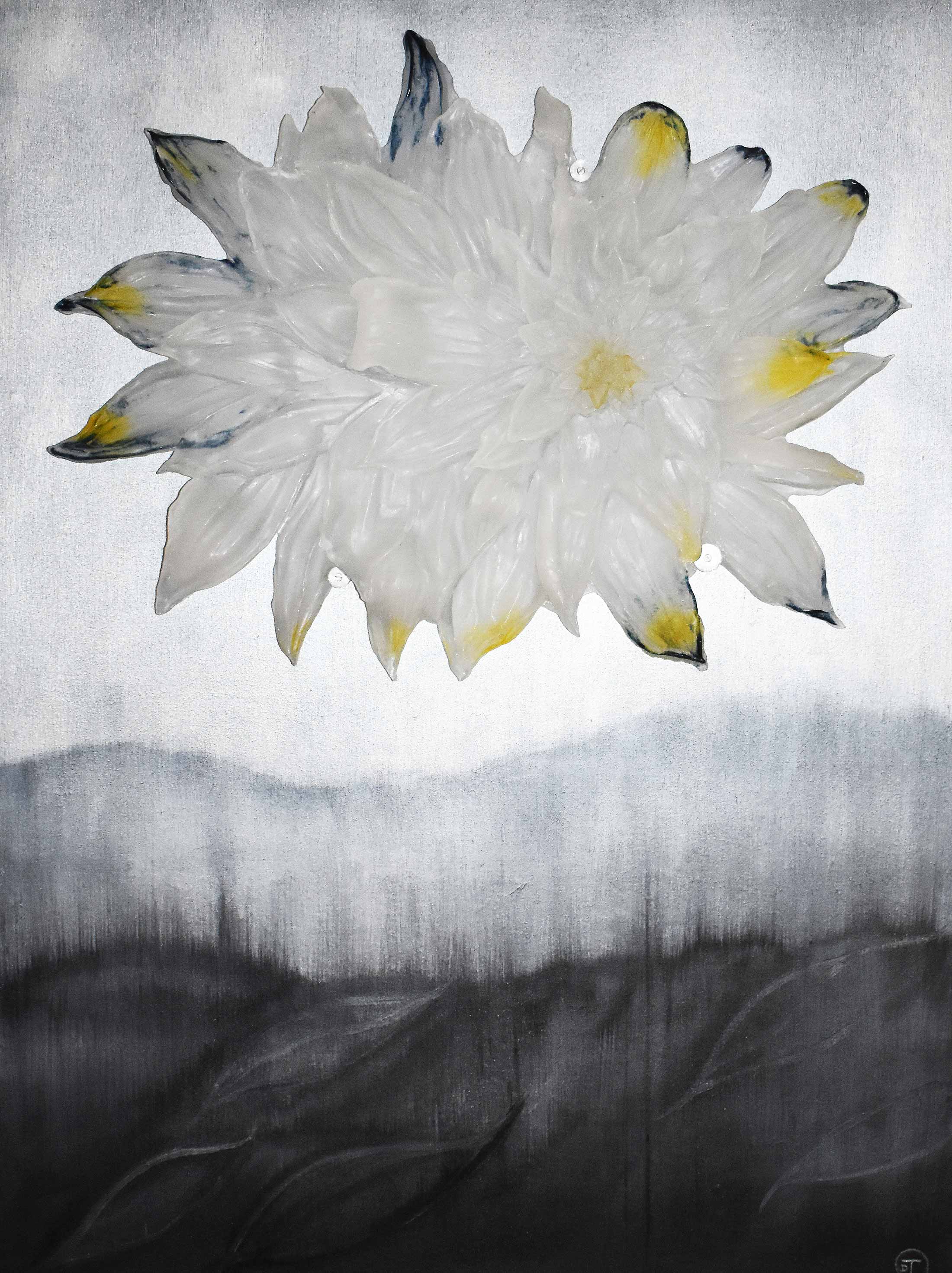The image is an intricate illustration or painting depicting two stylized flowers. The artwork features a layered background, transitioning from a dark black base at the bottom to a lighter grey and finally to a white section at the top. This gradation suggests a distant view with a wavy, staticky quality reminiscent of a seismograph's chart. The flowers, positioned centrally, are predominantly white with realistic petals that are intricately detailed, showcasing black and yellow borders. The flowers stand out against the abstract, textured background, evoking a sense of depth and dimensionality within the art piece.